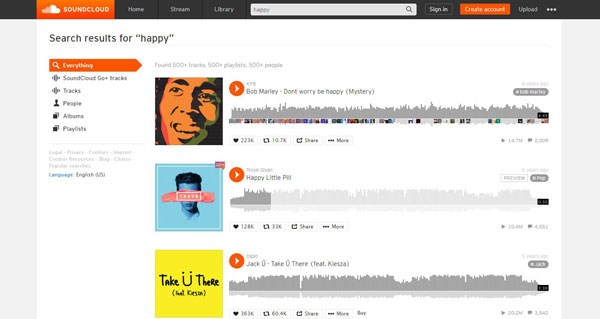An image displaying the SoundCloud user interface prominently showcases an orange bar at the top-left corner with navigation options like Home, Stream, and Library. In the center of the screen, a search query for "Happy" has been entered, resulting in numerous search results including tracks, people, albums, and playlists. The screen indicates a substantial amount of content with tags noting “500+ Tracks,” “500+ Playlists,” and “500+ People.”

Noteworthy search results include popular tracks such as "Don't Worry, Be Happy" by Bob Marley and "Happy Little Pill." Icons and tags accompany some tracks, showing they were uploaded approximately five years ago. Visual cues include an orange circle for tags and notable mention of specific playlists and users like "Take You There," "Jack," and "If You Dream, Consider."

A specific album catches the eye due to the blue background accented with red, with an artwork featuring Bob Marley's multi-colored faces—orange, red, and green—set against a contrasting background.

A Grade bar reflects user engagement metrics, highlighting "63,000 more" interactions and a notable "20.2." Overall, the interface maintains SoundCloud’s signature orange theme, enhancing the visual hierarchy and user navigation experience.